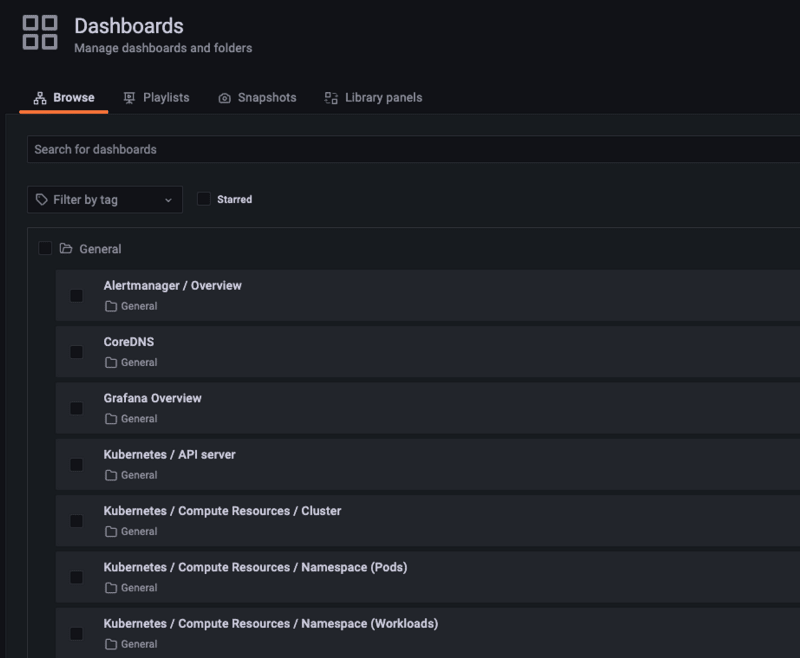The image features a black background with various UI elements organized in a structured layout. At the very top, there are four small gray boxes positioned together, labeled "Dashboards" and "Manage Dashboards and Folders". Below this, a navigation menu includes options such as "Browse" (which is underlined in red), "Playlists", "Snapshots", and "Library Panels".

Beneath the navigation menu, a prominent black search bar is labeled "Search for Dashboards". Adjacent to it, a box labeled "Filter by Tag" and another one labeled "Starred" can be seen. Below these elements, the word "General" marks the category for the listed items.

The main section contains several black boxes, each preceded by a smaller black sub-box, displaying titles of different dashboards. The first box is titled "Alert Manager Overview" and is categorized as "General". Following this, additional boxes are labeled: "Core DNS" (General), "Grafana Overview" (General), "Kubernetes API Server" (General), "Kubernetes Compute Resources and Cluster" (General), "Kubernetes Compute Resources, Namespace, Pods" (General), and "Kubernetes Compute Resources, Namespace, Workloads" (General).